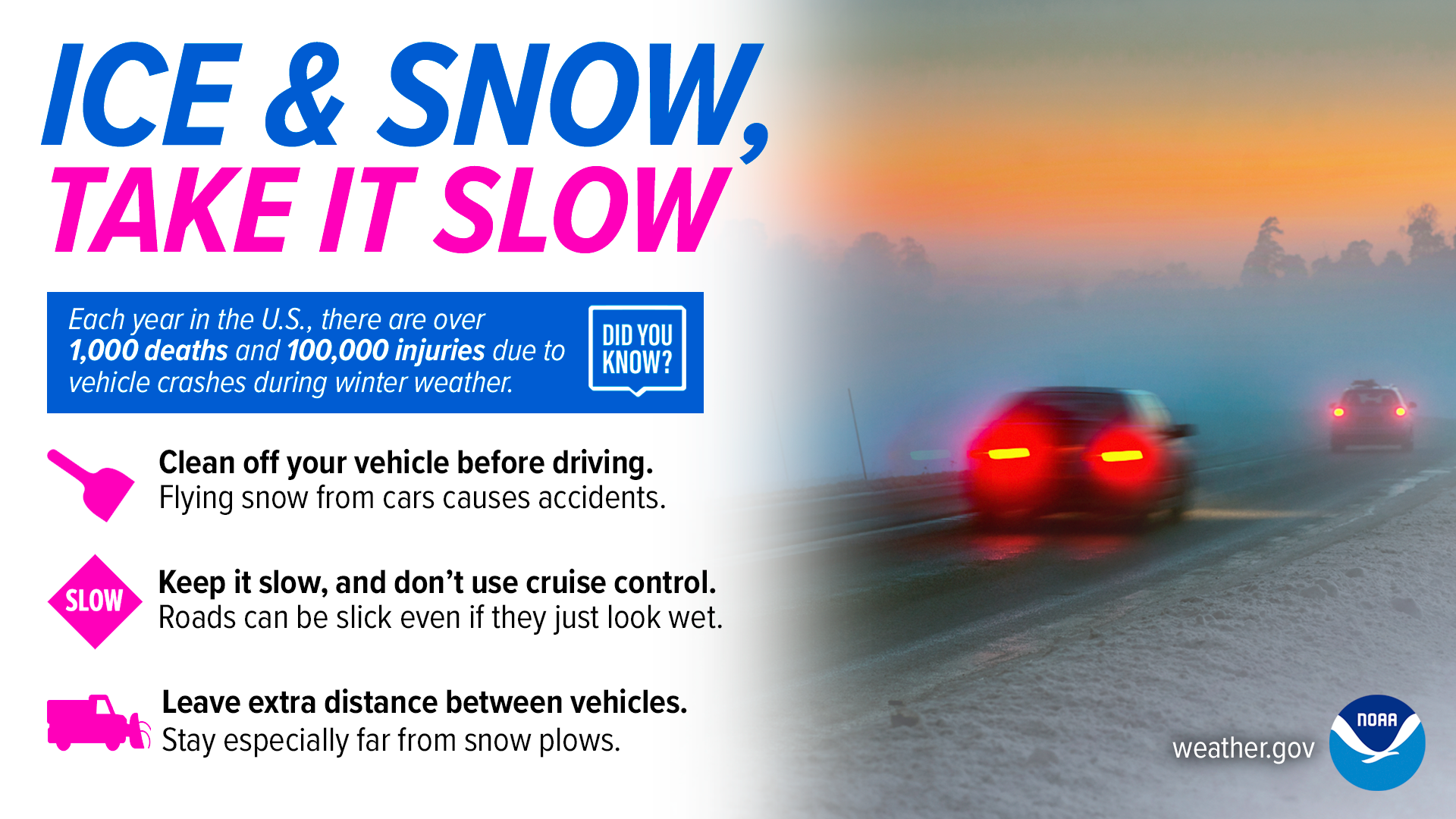The advertisement from weather.gov features a compelling and informative design to promote safe driving in winter conditions. On the left side, the heading "Ice and Snow – Take it Slow" is displayed prominently in blue and purple-pink text. Below this, a blue box highlights a sobering statistic in white lettering: "Each year in the U.S., there are over 1,000 deaths and 100,000 injuries due to vehicle crashes during winter weather." Adjacent to this, a white "Did You Know?" label catches the eye. 

Furthermore, a series of crucial safety tips are listed:
- "Clean off your vehicle before driving. Flying snow from cars causes accidents."
- "Keep it slow. Don’t use cruise control. Roads can be slick even if they just look wet."
- "Leave extra distance between vehicles. Stay especially far from snow plows."

The tips are visually supported by icons of a snow scraper, a "slow" stop sign, and a snow plow, each in pink.

On the right side of the advertisement, a hazy, snow-covered background features two cars traveling on a clear but icy road. Their taillights are illuminated, emphasizing the need for caution. The overall scene is captured in a muted, wintery palette, and the bottom right corner displays the weather.gov logo and the NOAA emblem, lending credibility to the message.